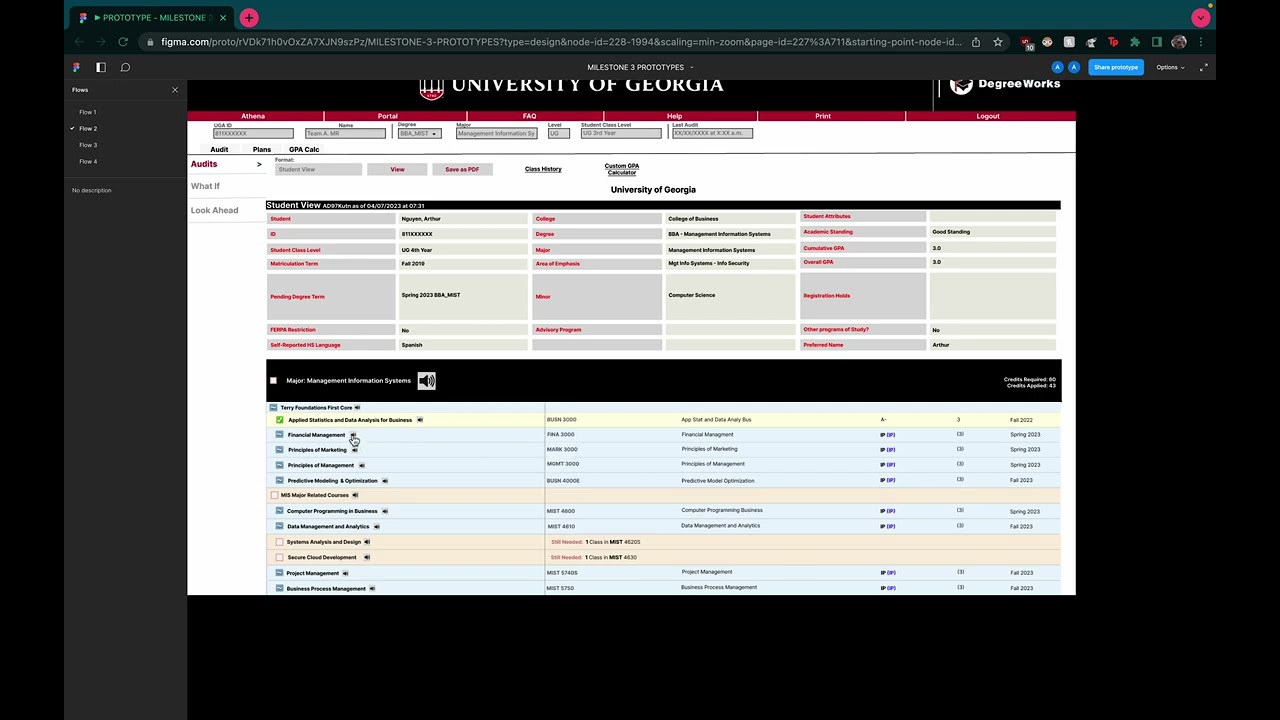This image is a screenshot of an open browser window displaying a prototype on Figma.com, specifically titled "Milestone 3". The prototype appears to be a web portal for the University of Georgia. The URL in the address bar confirms the Figma platform, used for collaborative design. The screen is divided by a prominent black horizontal bar separating two main sections of content. 

At the top, a header with a black background and white University of Georgia text stands out. Below this, the central part of the prototype includes six columns in pastel colors—green, blue, and pink—containing various data. The left side of the interface shows a navigation menu with options such as "audits," "what if," and "look ahead," with "audits" being the active link. The right side of the main body prominently features a "student view" section, which includes a table of student-related data. 

There are Figma UI elements visible, including a side panel labeled "Flows" with Flow 2 currently selected out of four available flows. The resolution of the text is slightly unclear, indicating the need for zooming in to read specific details. The entire design reflects a work-in-progress portal aimed to provide students with access to their GPAs, attributes, and potentially other academic-related information, suggesting possible future use by teachers as well.